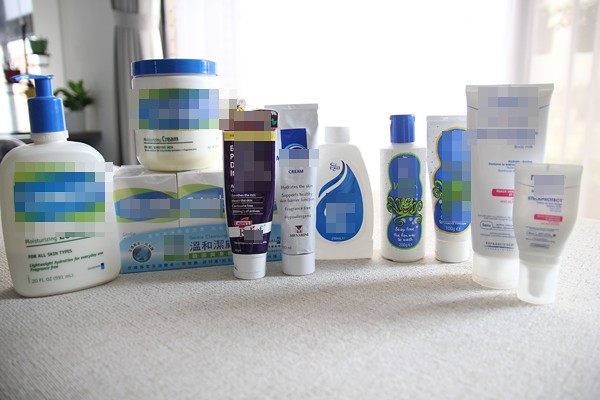The image features an array of skincare products meticulously arranged on a countertop adorned with a fabric tablecloth. Though the labels are pixelated, the bottle shapes and color patterns hint that these are predominantly from the Cetaphil brand, characterized by their white bottles and blue text. The items, varying in types, are neatly organized across the table, showcasing a comprehensive skincare routine. In the blurry background, gray curtains tied to the side can be seen, alongside a delicate, gossamer-like white curtain on the left, adding a soft texture to the setting.